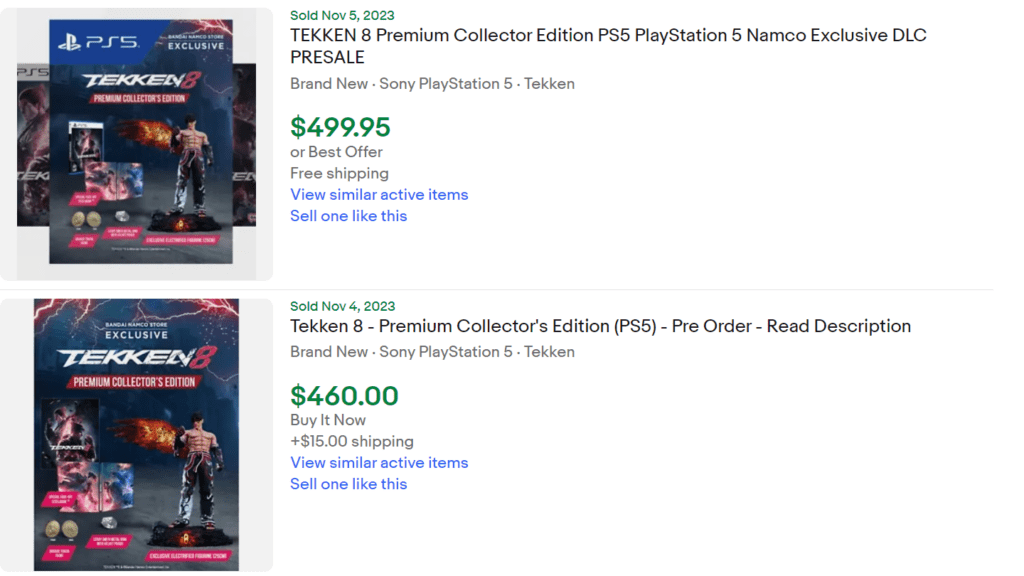The image is a screen grab of two payment options for Tekken 8 displayed on a plain white background. The screen is divided into two sections, top and bottom. In the upper section, on the left, it features a PS5 Exclusive Tekken 8 Premium Collector's Edition title with an accompanying image of a character from Tekken 8 adorned with fiery wings. Additional imagery is also present. To the right in this section, green text indicates "Sold November 5th, 2023." Below this, it reads "Tekken 8 Premium Collector's Edition PS5 PlayStation 5 Namco Exclusive DLC Presale," followed by "Brand New Sony PlayStation Tekken." The price is listed in green as "$499.95," and in gray text, it offers "Or Best Offer Free Shipping." There is also a blue hyperlink stating "View Similar Active Items or Sell One Like This."

In the lower section, the left side mirrors the imagery of the top section but without the PS5 logo. It reads "Exclusive Tekken 8 Premium Collector's Edition" with similar icons. On the right, green text indicates "Sold November 4th, 2023." Beneath this, in black, it states "Tekken 8 Premium Collector's Edition PS5 Pre-Order Read Description," followed by "Brand New Sony PlayStation 5 Tekken." The price here is "$460" in green, with "Buy It Now Plus $15 Shipping" in gray below. A blue hyperlink follows, reading "View Similar Active Items, Sell One Like This."